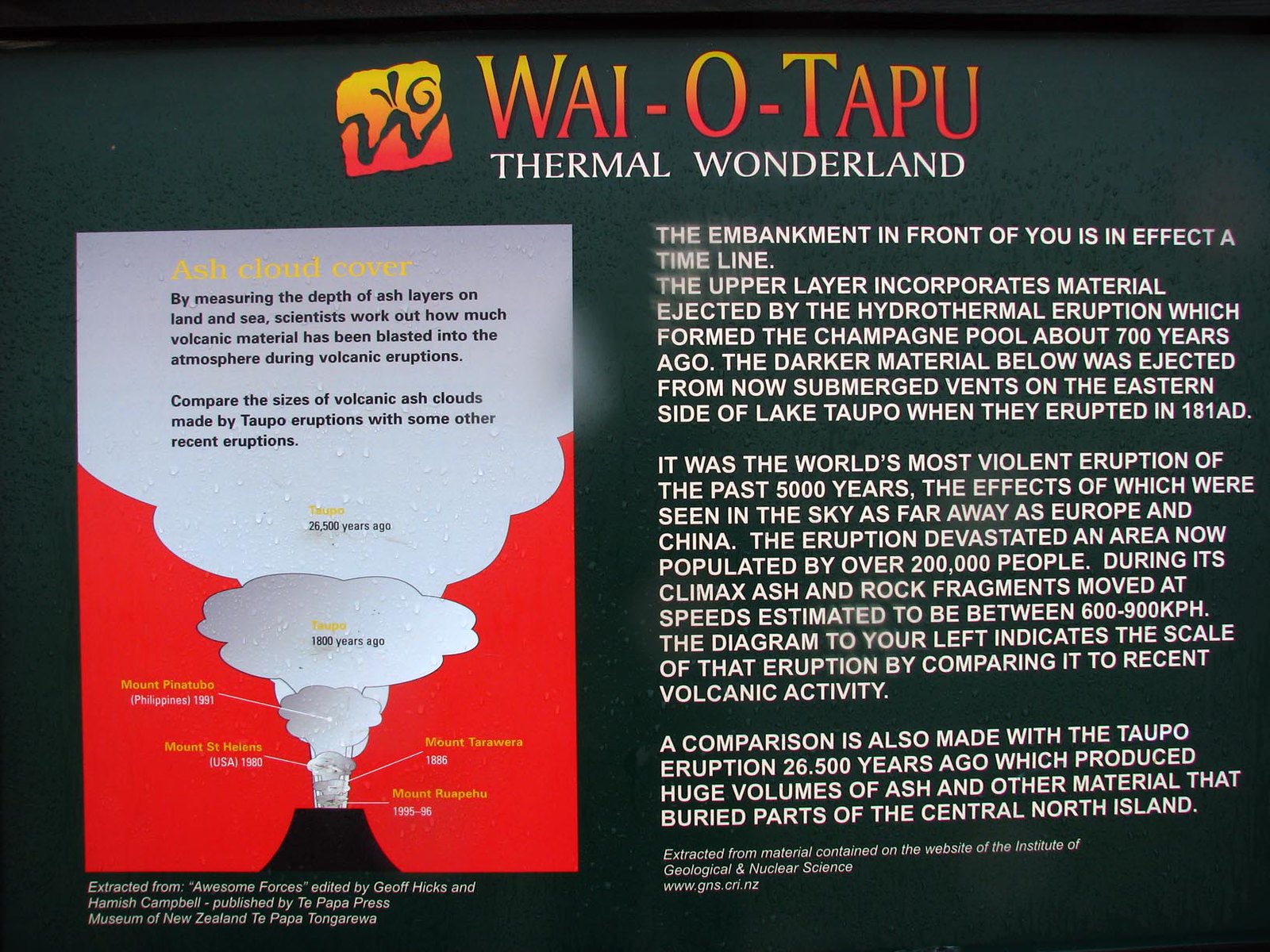This is an informative sign with a dark gray or black background, prominently titled "Wai-O-Tapu" at the top in bold letters, with a gradient from yellow at the top to red at the bottom. Adjacent to the title is a square logo in red and yellow featuring a large 'W'. Below it, the sign reads "Thermal Wonderland" in all caps, white letters. 

On the left side of the sign, there is a vertical diagram with the header "Ash Cloud Cover". This section explains in detail how scientists measure the depth of ash layers on land and sea to estimate the volume of volcanic matter ejected during eruptions. The diagram compares the sizes of volcanic ash clouds from the Taupo volcanic events with recent eruptions, including timelines such as 26,000 years ago and 1,800 years ago. At the bottom, it credits the information to "Awesome Forces" edited by Jeff Hicks and Hamish Campbell, published by Te Papa Press, Museum of New Zealand Te Papa Tongarewa.

On the right side, there are three paragraphs of text in white letters, aligned to the left. The text describes how the embankment in front of the viewer serves as a natural timeline. It explains that the upper layer consists of material ejected by the hydrothermal eruption which formed the Champagne Pool approximately 700 years ago. The deeper, darker layer was expelled from now-submerged vents on the eastern side of Lake Taupo during an eruption in 181 AD, noted to be the most violent in the past 5,000 years. The effects of this eruption were seen as far away as Europe and China, devastating an area currently inhabited by over 200,000 people, with ash and rock fragments propelling at speeds estimated between 600 and 900 kph. The diagram to the left illustrates the scale of this eruption in comparison to more recent volcanic activity and the massive Taupo eruption 26,500 years ago.